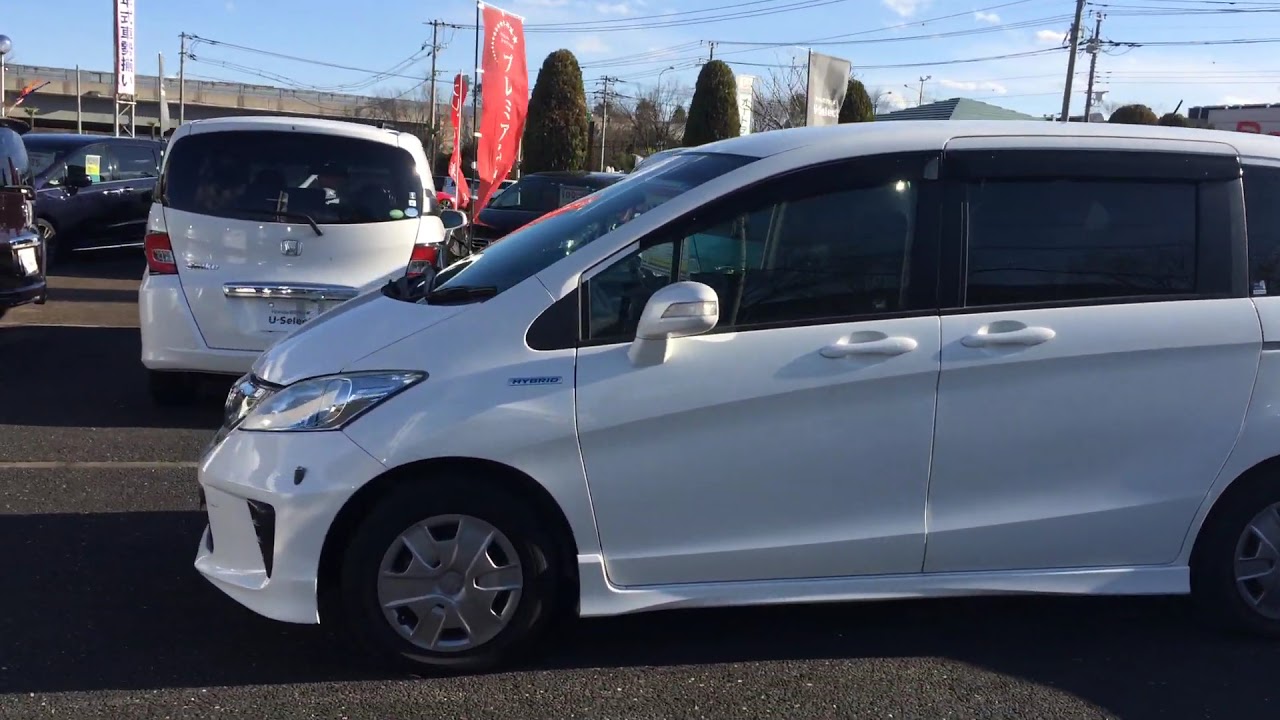In this image, we observe an outdoor scene likely set in a car dealership in the middle of the day. Dominating the center is a reflective silver or white hybrid van, seen from the side with clear views of the driver's side and part of the passenger door, as well as its wheels. The van is parked sideways on an asphalt surface marked with white parking lines. Surrounding the main vehicle, there are numerous other cars, including white and black models, neatly lined up in the parking lot.

In the midground, we spot more cars, some of which bear Hyundai logos, suggesting this could be a Hyundai dealership. Red banners with Asian writing add a distinctive touch to the background scene. Additional details include trees, an overbridge, telephone poles, and electric wires prominently silhouetted against the clear daytime sky.

This detailed visual showcases hues of black, gray, silver, white, red, green, blue, and orange, contributing to a vivid capture of this automobile-filled, urban environment.